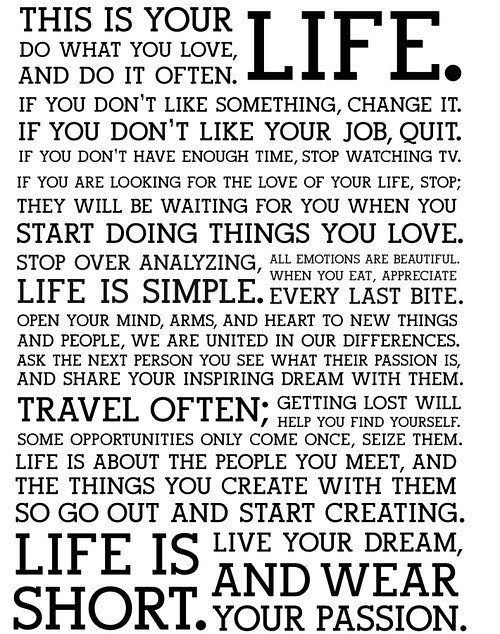The image has a white background with varying sizes and boldness of black text, stretching from the top left to the bottom right. It begins with the prominent phrase "This is your life." in large letters. The text encourages: "Do what you love and do it often. If you don't like something, change it. If you don't like your job, quit. If you don't have enough time, stop watching TV. If you are looking for the love of your life, stop. They will be waiting for you when you start doing things you love. Stop overanalyzing. All emotions are beautiful." 

It continues with: "Life is simple. When you eat, appreciate every last bite. Open your mind, arms, and heart to new things and people. We are united in our differences. Ask the next person you see what their passion is and share your inspiring dream with them. Travel often. Getting lost will help you find yourself. Some opportunities only come once. Seize them." 

The text concludes with: "Life is about the people you meet and the things you create with them, so go out and start creating. Life is short. Live your dream and wear your passion."